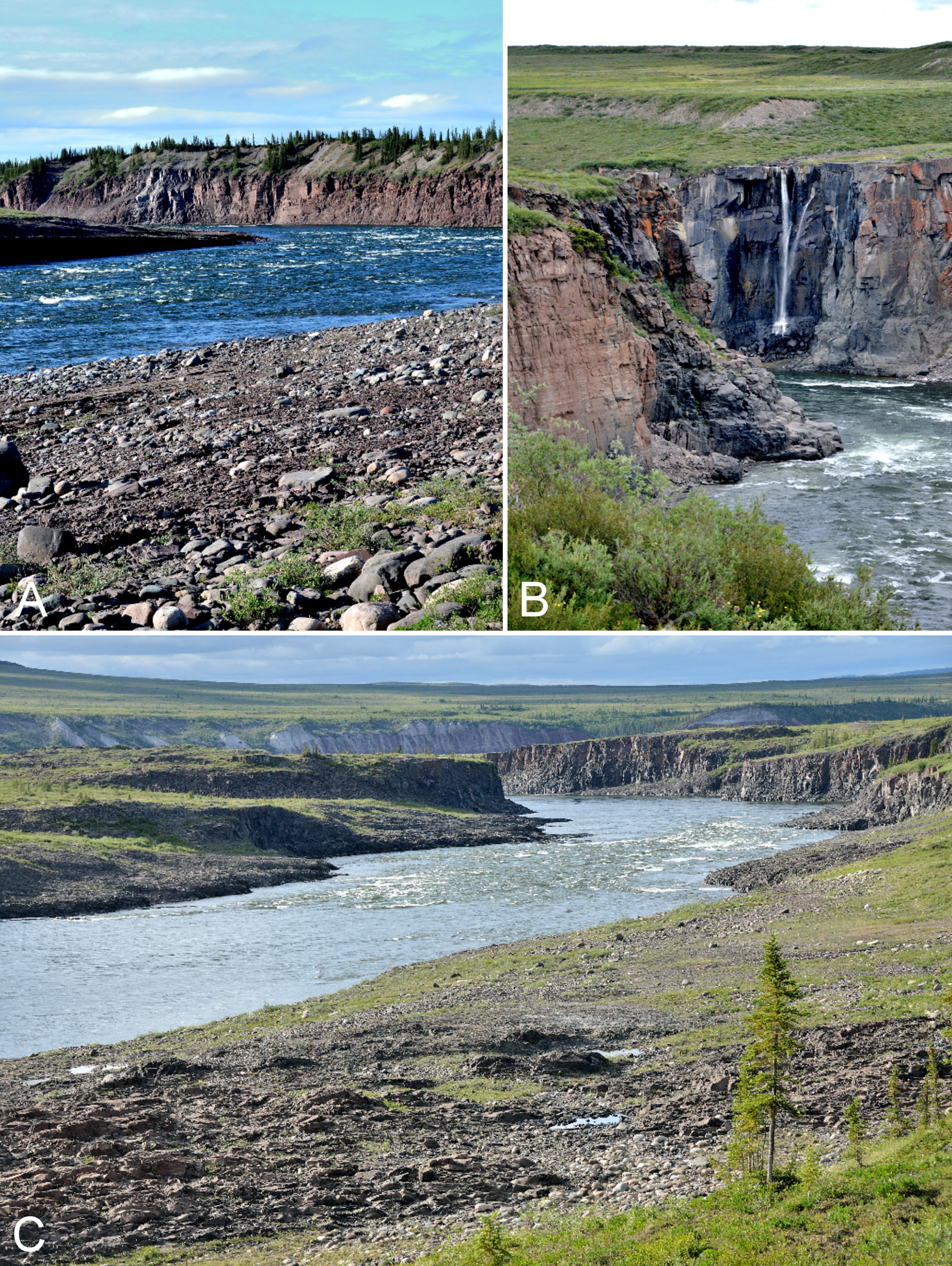The collage consists of three labeled photographs, A, B, and C, showcasing breathtaking landscapes with water and rocky terrains. In the top left image (A), there is a striking view of the dark blue ocean, bordered by rugged, dark gray rocks. This scene is set against the backdrop of a stone-like hill covered in lush grass and trees. The top right image (B) features a majestic cliff with a waterfall cascading down, surrounded by green grass atop dark gray rock formations, and below, a large body of dull teal water. This image also includes bushes on the left side. The bottom photograph (C) captures a river with water flowing towards the center of the frame, flanked by masses of land that are a mix of grass and rocky areas. Notably, a green tree appears in the bottom right corner of this image. The vivid and varied hues of blue water in these photographs range from the dark blue ocean in A to the lighter blue of the river in C, creating a harmonious yet diverse visual narrative.